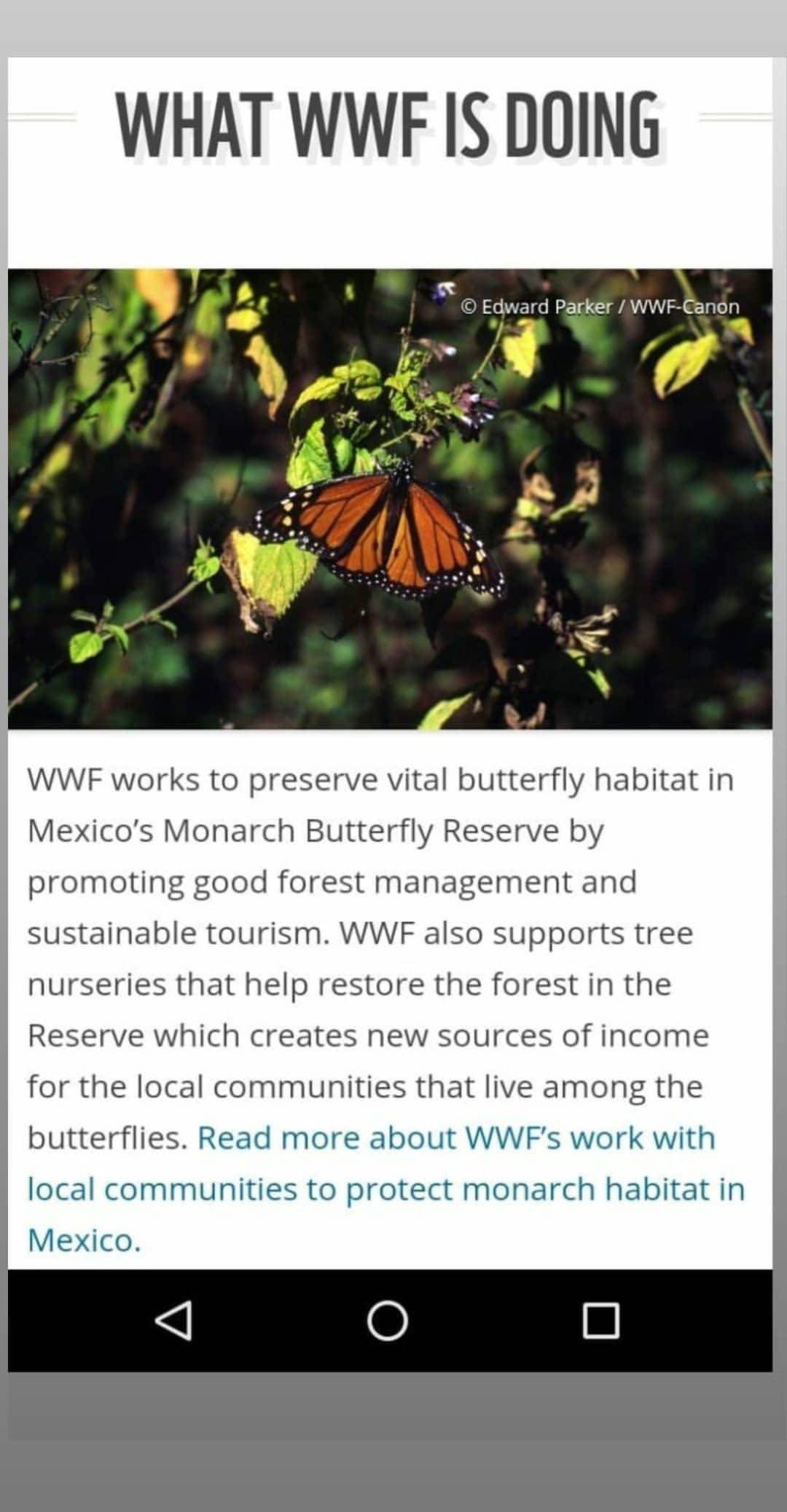This image captures a computer screen displaying a web page about the World Wildlife Fund (WWF) and its efforts with monarch butterflies. Dominating the page is an elegant photograph of a monarch butterfly resting amidst tree branches. Below the image, the text reads, "What WWF is doing?" The detailed description underneath reveals that the WWF is dedicated to preserving butterfly habitats in Mexico's Monarch Butterfly Reserve. Their initiatives include promoting sustainable tourism and good forest management practices. Additionally, WWF supports local tree nurseries to restore forest areas within the reserve, creating new income opportunities for local communities coexisting with the butterflies. The photo is credited to Edward Parker/WWF-Canon.

Further down the page, a section highlighted in blue invites viewers to "read more about WWF's work with local communities to protect monarch habitat in Mexico." At the bottom of the screen, there is a user interface section with a black rectangle housing white icons for a triangle, a circle, and a square, likely representing media player controls or navigation buttons.